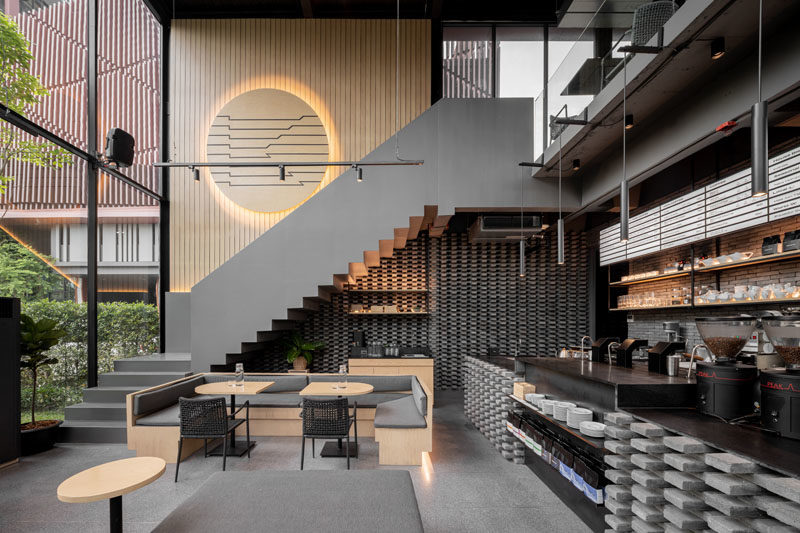The image depicts the interior of a modern, predominantly gray, two-story coffee bar or café with a stylish and minimalist design. The space features grid-like counters made from spaced-out cinder blocks, contributing to its industrial chic vibe. A striking centerpiece is the gray staircase in the back, leading to an upper level, which accompanies the sleek circular light fixture. The walls showcase straight wooden paneling with a sun or moon design cut into them, accentuated by subtle backlighting.

At the forefront, there is a seating area furnished with gray cushioned booths and black chairs, exemplifying the establishment's muted aesthetic. Additional seating includes tables with black chairs and a booth with gray cushions and a wooden base. Cylindrical lights suspended from the ceiling illuminate this area.

The coffee bar itself is crafted from gray concrete, with metal faucets and various containers—large vats and conical upside-down ones—positioned along the counter for serving beverages. Shelves stocked with cups and a coffee grinder suggest a focus on coffee, though the presence of other containers hints at tea service as well. Behind the counter, there is a white menu displayed in a grid format with black lettering.

The establishment is characterized by modern elegance with a checkerboard pattern of protruding stones on the wall adding texture, and large windows offering views of greenery outside, enhancing the peaceful ambiance.